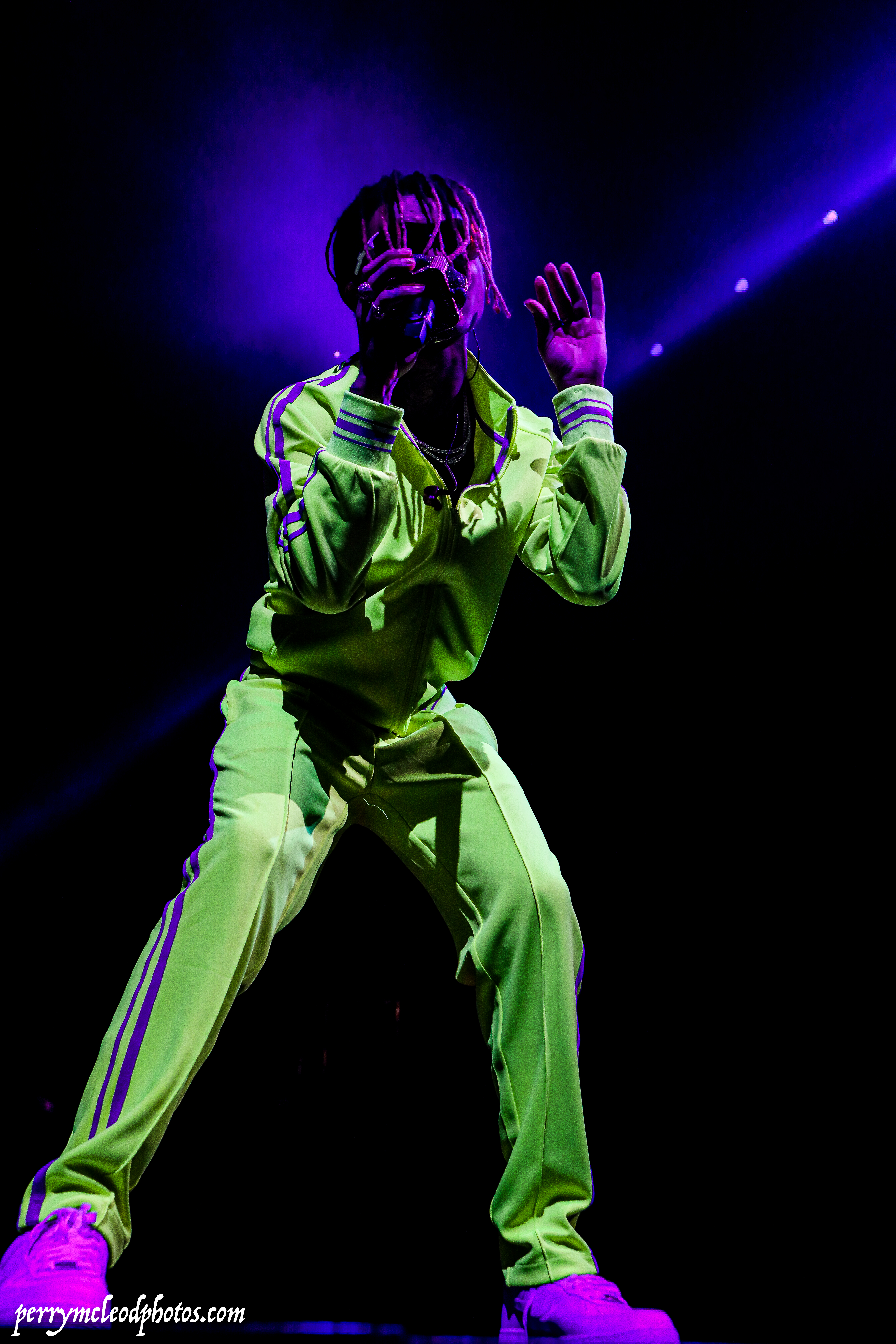This is a photograph capturing a man possibly performing on a stage, his figure illuminated by vibrant blue and purple spotlights against a black backdrop. He appears to be wearing a neon green tracksuit with bold purple vertical stripes running down the sleeves of the jacket and the pant legs. His face and sneakers, also glowing in neon purple hues, highlight the intensity of the lighting. The man is bending over slightly with his hands raised in front of his face. The bottom-left corner of the image features the italicized white URL, perrymccleedphotos.com, written entirely in lowercase letters.